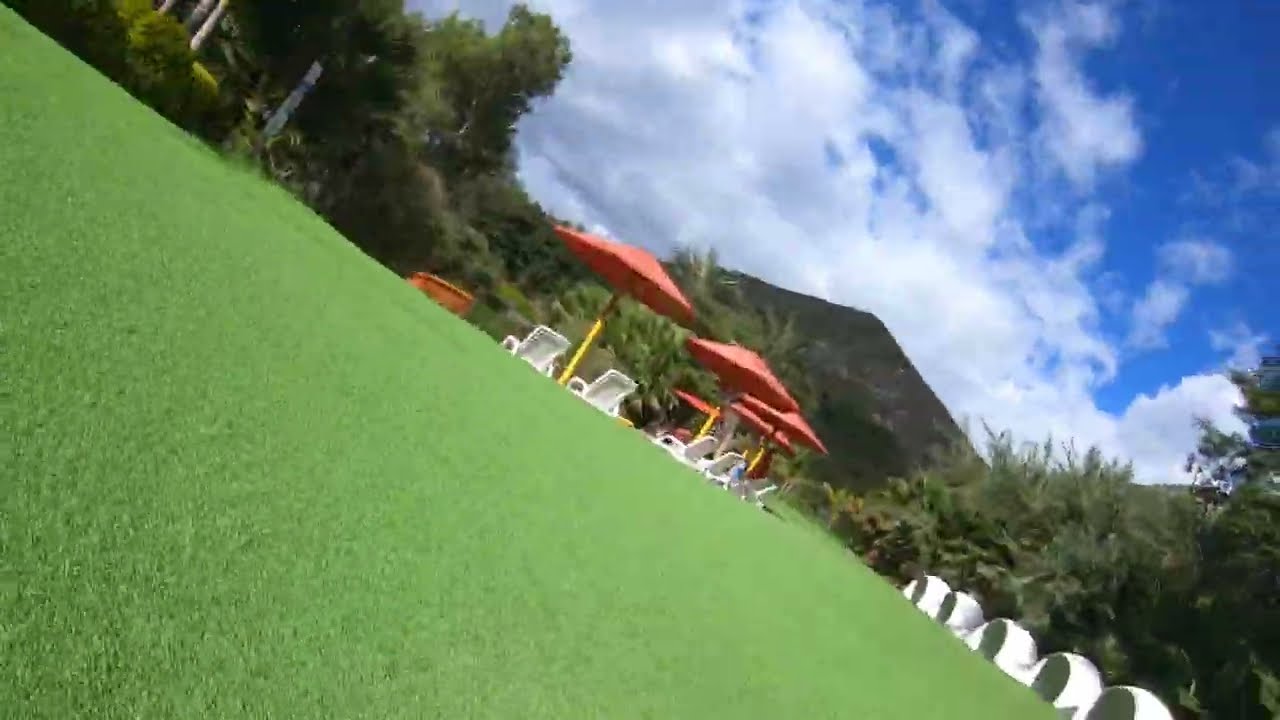The photograph, taken from a low vantage point and slightly tilted, captures a vibrant garden scene. Dominated by bright green grass in the foreground, a row of white plastic lawn chairs are strategically arranged, with each pair shaded by a red sun umbrella supported by a yellow pole. Approximately four or five umbrellas can be seen. Enclosing the garden are lush, fluffy green trees and some green shrubs. To the bottom right of the image, white circular objects are partially visible. Beyond the garden's edges, tall trees frame the view, and a triangular, brownish-green hill rises in the distance. The sky above is a vivid blue, adorned with large, white clouds. The entire scene is bathed in bright daylight, emphasizing the vivid colors and lively atmosphere.